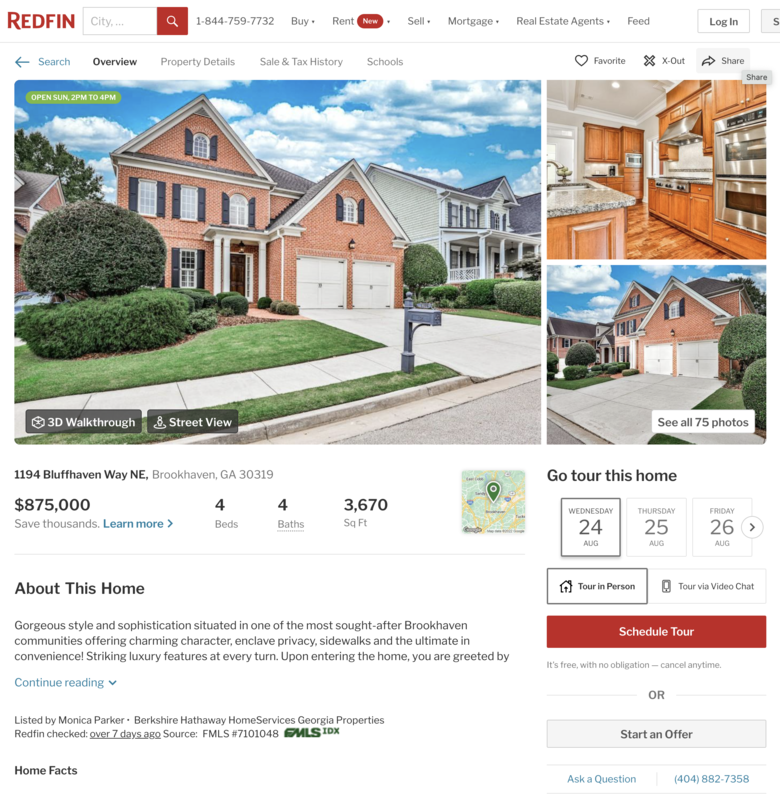A screenshot of a property listing on Redfin showcases a well-organized interface with a white background and dark gray text, accentuated by red and blue elements. The Redfin logo is prominently situated in the top left corner. A search bar partially visible reads 'city', and a customer service phone number, 1-844-759-7732, is displayed. The top navigation bar provides links titled 'Buy', 'Rent' (marked as new with a red oval and white text), 'Sell', 'Mortgage', 'Real Estate Agents', and 'Feed'. Buttons for login and sign-up are also present but partially cut off.

The listing features professional, brightly-lit photographs of a large, brick house in a pristine neighborhood. The home, located at 1194 Bluff Haven Way NE, Brookhaven, Georgia, 30319, is priced at $875,000 and boasts 4 bedrooms, 4 bathrooms, and spans 3,670 square feet. Detailed home information is provided below the photos, along with options to schedule a tour, start an offer, ask a question, or contact the agent directly at 404-882-7358. The meticulous landscaping and well-maintained surroundings are highlighted, giving a sense of the property's high quality and desirability.